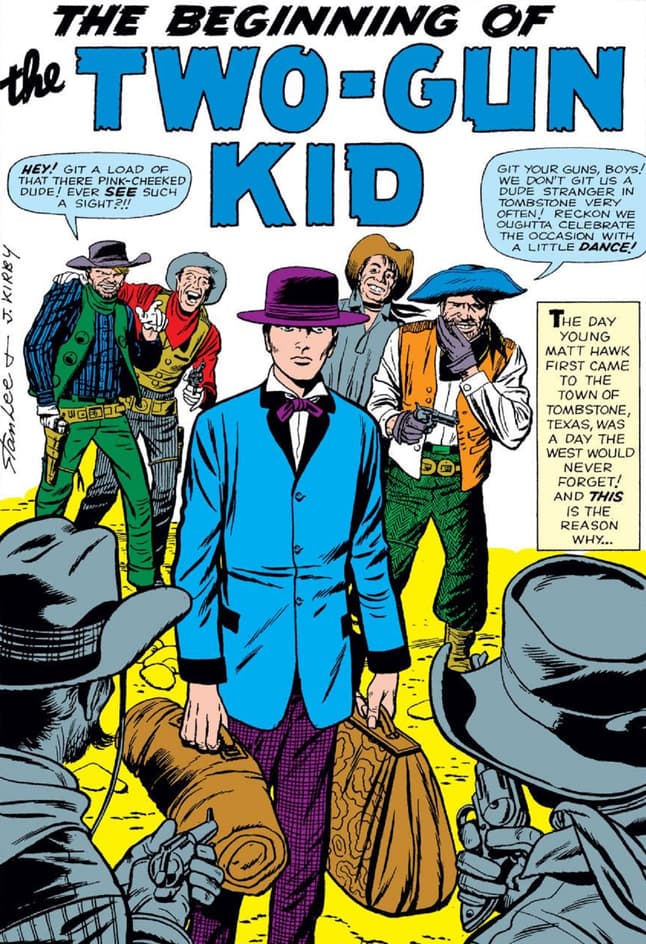The image is a cartoon-style comic book cover titled "The Beginning of the Two-Gun Kid." It features a young man, Matt Hawk, in the center, dressed in a blue suit with black-edged sleeves, a white shirt, a purple bow tie, purple hat, and purple pants. He holds a carpetbag in his left hand and a rolled-up sack in his right. Surrounding him are several cowboys, adding tension to the scene. 

To Matt's left and right, two cowboys with guns drawn aim at him. The cowboy to his left is in a green outfit with a hand on a holstered gun, alongside another cowboy in a brown vest and red shirt, laughing. The man in green addresses Matt with a speech bubble saying, "Hey, get a load of that there pink cheeked dude. Ever see such a sight?" To Matt's right, another cowboy smiles while wearing a gray shirt and brown hat, standing next to a man in an orange vest, white shirt, green pants, brown boots, and a white-brimmed hat who says, "Get your guns boys, we don't get a dude stranger in Tombstone very often. Reckon we're gonna celebrate this occasion with a little dance."

Above the cowboys, the title in black text reads "The Beginning of the Two-Gun Kid," with "The Two-Gun Kid" in blue. Below, a caption box narrates, "The day young Matt Hawk first came to the town of Tombstone, Texas was the day the West would never forget—and this is the reason why." At the far left, the names "Stan Lee" and "Jack Kirby" appear. The ground beneath them is yellow, adding contrast to the vivid character designs and text.